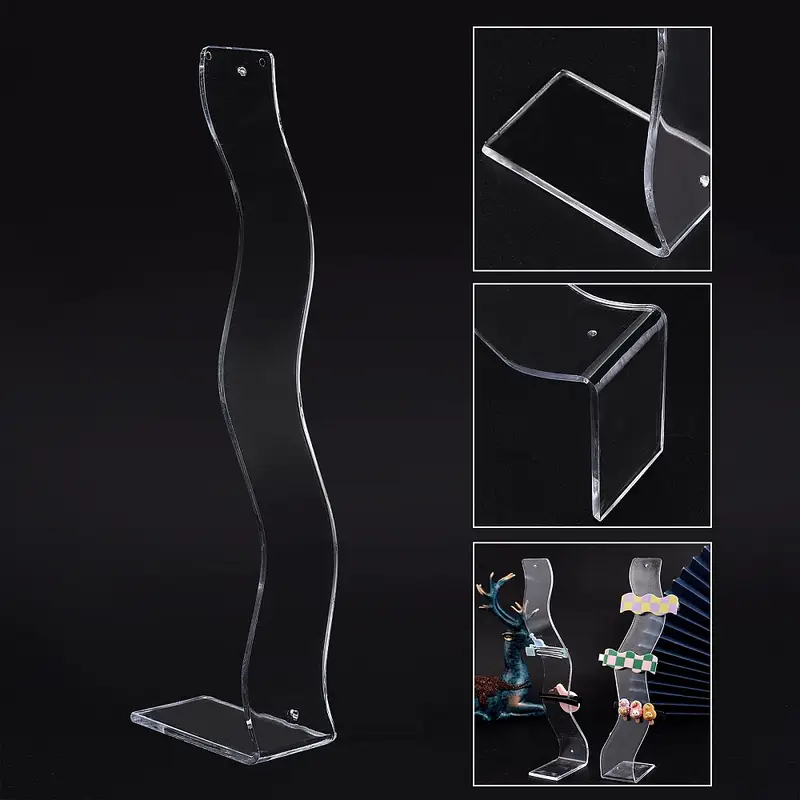The image features a glass-like, curvy, rectangular-stemmed stand on the left side, extending from the top to the bottom of the frame. This transparent plexiglass stand has an undulating stem with distinct holes at the top and bottom. To the right, three segmented box images provide detailed views of the stand. The top box offers a close-up of the stand's base, while the middle box shows the stand lying down, detached from the platform. The bottom box displays two decorated glass stands, suggesting possible uses for holding items like colorful hair clips in checkerboard patterns of green and white or purple and yellow. The solid black background accentuates the vivid blue deer with yellow antlers and a brown object, alongside a blue hand fan-like pattern on the right.